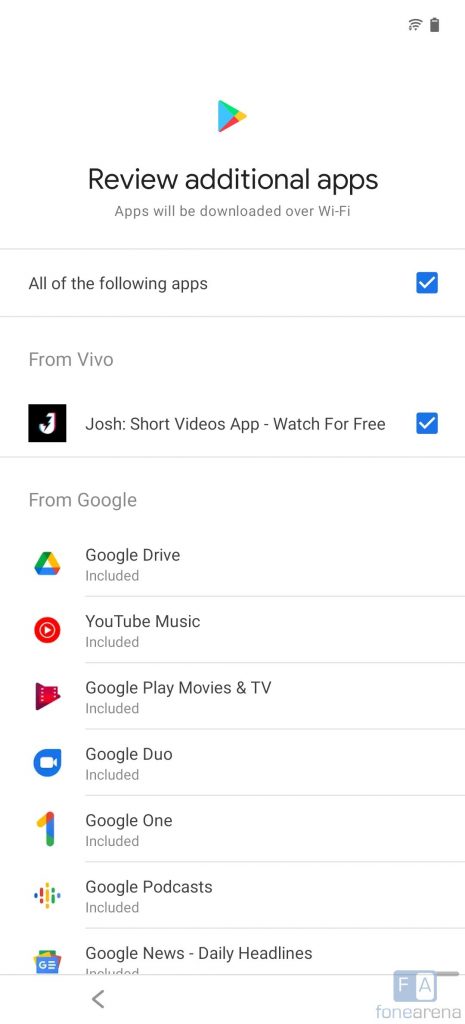The image is a screenshot from a smartphone displaying a list of applications available on the Google Play Store. The top section of the screenshot shows the phone’s status bar, including battery and Wi-Fi indicators. Below the status bar, there is a title stating "Review additional apps. Apps will be downloaded over Wi-Fi" along with the Google Play Store logo.

The list of applications is categorized as follows:

- The first section is labeled "From Vivo" and includes an app named "Josh - Short video apps, watch for free," with the selection box checked.
  
- The second section is labeled "From Google," featuring a series of pre-included apps:
  - Google Drive (Included)
  - YouTube Music (Included)
  - Google Play Movies & TV (Included)
  - Google Duo (Included)
  - Google One (Included)
  - Google Podcasts (Included)
  - Google News - Daily Headlines (Included)

At the bottom of the screen, a back button is visible, allowing the user to navigate back to the previous menu. Additionally, a watermark reading "Phone Arena FA" is situated at the bottom of the image, indicating the source of the screenshot.